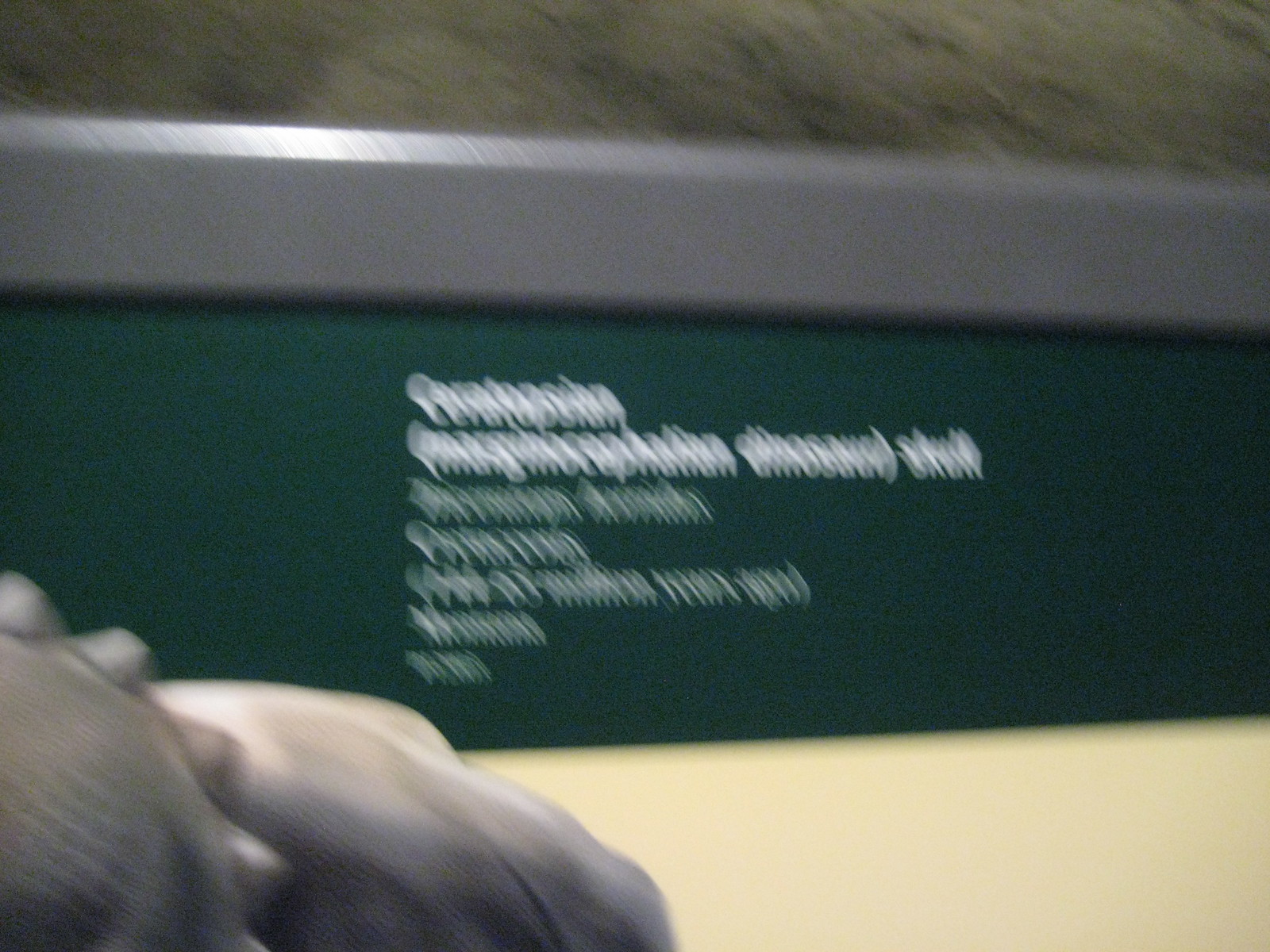A blurry image captures a scene with a variety of textures and colors. The primary background is a gray carpet, providing a muted backdrop. At the center of the image is a transparent plastic square frame, superimposed on a dark lawn green surface. The green background inside the frame features white lettering, but the text is too blurred to decipher and appears to be in an unfamiliar language. In the bottom left corner of the image is a gray arm, adorned with a rounded sun-spike motif. To the right of the frame, the background transitions into a plain vanilla color, devoid of any writing or distinguishing marks. Overall, the image is too unfocused and grainy to capture any significant details, leaving only a vague impression of the objects and text within it.